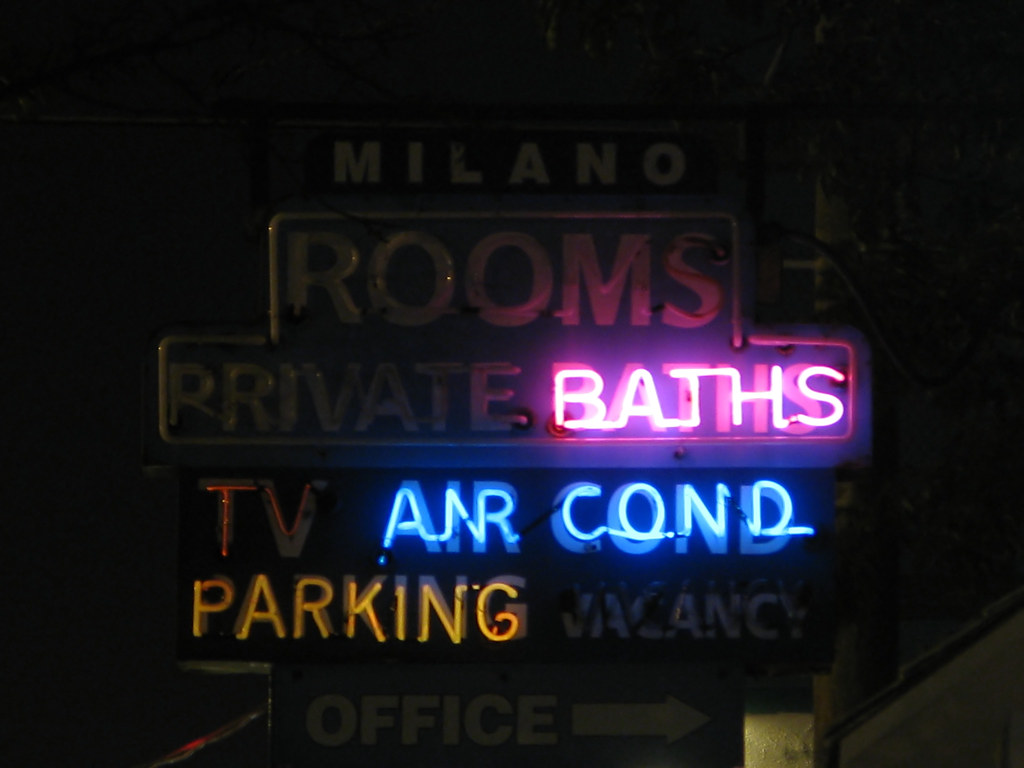This is a detailed nighttime photograph featuring a partially illuminated neon sign for a hotel. The sign reads "Milano" at the top, followed by "Rooms," "Private Baths," and various amenities like "TV," "Air Con," "Parking," "Vacancy," and "Office," with an arrow pointing direction. The only letters lit up in the darkness are "Baths" glowing in pink, "Air Con" in blue, and "Parking" in yellow. All other sections of the sign remain dark, either turned off or burnt out. The photo is sharply focused on the glowing neon against a pitch-black background, with no additional lighting or visible details in either the foreground or background. The image captures the bright, glowing quality of the neon against the night sky, emphasizing the dim, partial lighting of the sign.